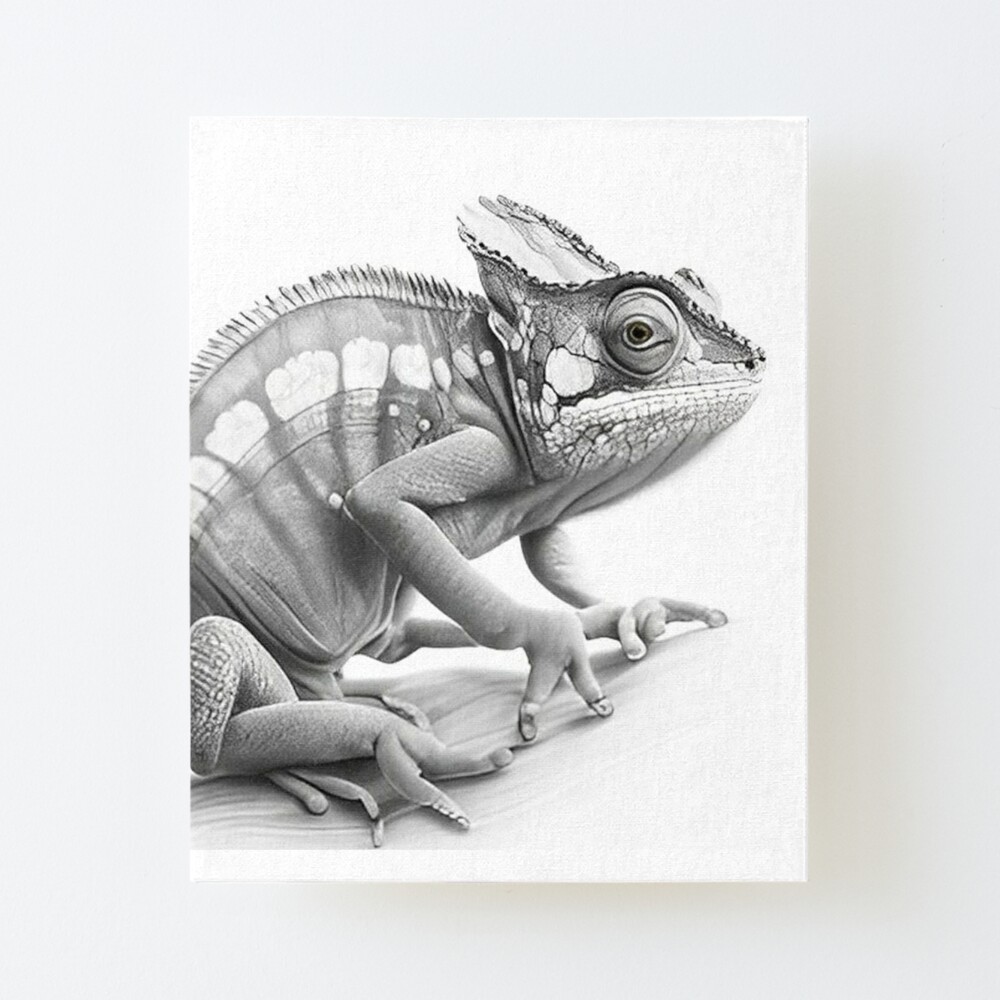This is a detailed, hand-drawn, black and white pencil illustration of a chameleon in profile facing right on a white canvas background. The chameleon is meticulously depicted with a series of light and heavy pencil strokes, giving it a photorealistic appearance. The chameleon's body features typical lizard skin patterns with white spots running down one visible side. It has prominent bulging eyes, with one staring directly at the viewer, and pointy ears. Its neck underneath the chin appears sagging and loose, consistent with a relaxed posture. The chameleon's legs are positioned so that the front feet and back feet are on the ground, with its tail intricately wrapped around its hind legs. A row of sharp, spine-like scales runs down the center of its back, adding a dinosaur-like quality to the creature. Each front hand, or leg, has distinctive three fingers, showcasing the intricacy of the drawing.